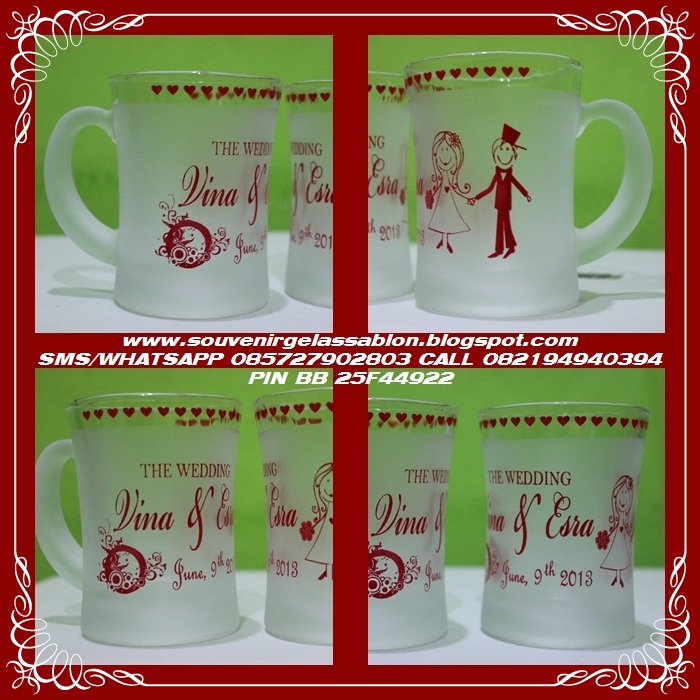This image is a detailed advertisement showcasing custom imprinted glass mugs designed for weddings or special occasions. The square format picture features four distinct sections, created by a red border with intersecting horizontal and vertical red stripes dividing the image into four quadrants. Each quadrant displays different views of frosted glass mugs with handles.

The mugs have a unique design: an unfrosted band decorated with red hearts along the top rim and intricate stick figure drawings depicting a bride and groom, accompanied by flowers, within the frosted section. The text on the mugs reads "Avina and Ezra, The Wedding, June 9th, 2013," all in red font.

In the center of the image, prominently displayed in white script, is the URL "www.souvenirglassesablanc.blogspot.com." Below the URL, additional contact information is provided, including WhatsApp and phone numbers, as well as a pin code.

The background combines photographic realism with graphic design and typography, portraying a professional and visually appealing advertisement. The blend of light green and white background colors, along with the red and white border, accentuates the custom wedding mugs effectively, emphasizing this as a promotional image for a company specializing in personalized glassware.